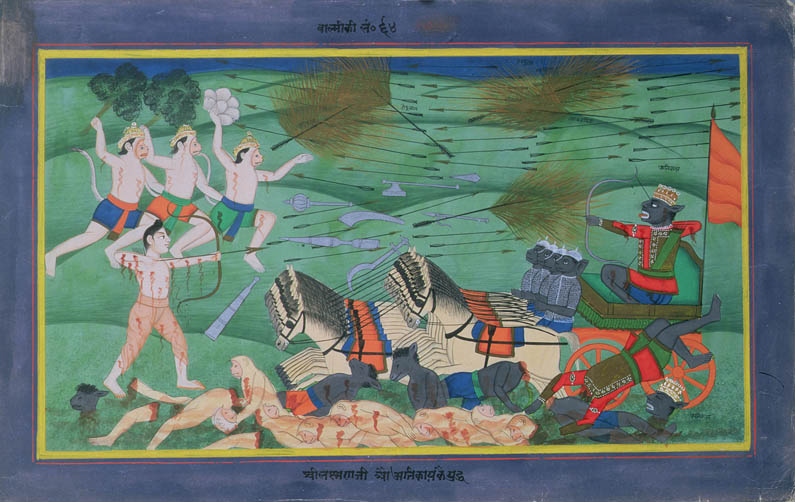The artwork features a meticulously detailed drawing encased in a purplish frame that adds an elegant touch to the composition. Within this frame, a yellow line emerges, intruding slightly into the drawing itself. The central focus is a man positioned in a chariot, firmly gripping a bow and arrow, poised as if caught in a moment of intense action. 

The chariot is drawn by two rows of horses, each row driven by four individuals who appear to be guiding the powerful creatures with precision. The scene unfolds dramatically at the base of the image, where bodies are strewn, suggesting a battlefield littered with the fallen.

In a chaotic flurry of movement, additional figures aim bows and arrows and hurl white circular objects towards the man in the chariot, adding to the sense of turmoil and conflict captured in this vivid piece of artwork.